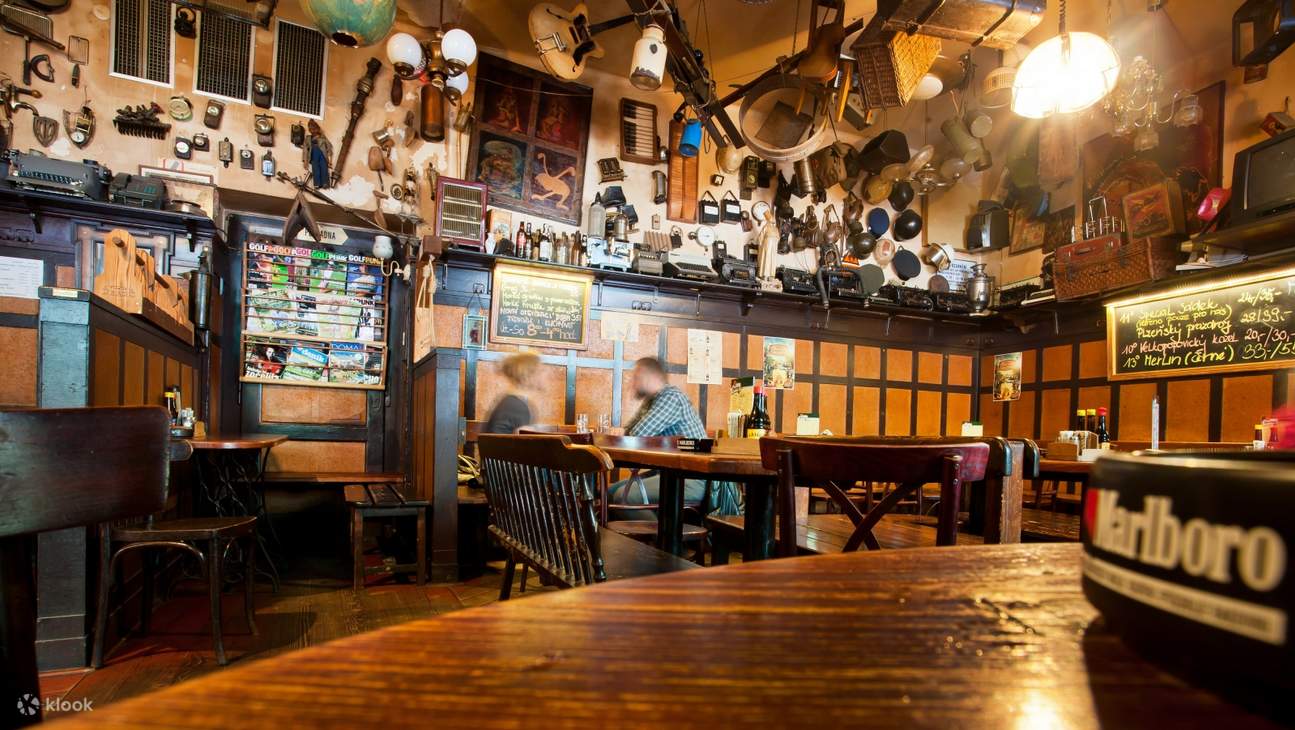The image depicts the cozy interior of a rustic-themed sports bar or tavern. The setting features wood paneling with a beige section rising above it, contributing to its warm, inviting ambiance. The walls are adorned with an eclectic array of western-themed gadgets and knickknacks, including baseball helmets, lanterns, and guitars. The ceiling is cluttered with baskets, pendant lights, illuminated mainly from the right, suitcases, lanterns, keyboards, pots, pans, and globe models of the earth.

In the foreground, there is a round oak table with a slightly blurred Marlboro ashtray placed near its edge. A black sign with white lettering displaying the Marlboro logo is also visible. Adjacent to this table is a red oak chair. The background reveals a couple sitting at a table with their faces blurred, near which a chalkboard marquee lists the day's specials and drinks. Behind them is the edge of a bar, with several tables and chairs placed around it.

Additional details include a brown, dark wooden shelf topped with typewriters, a radiator heater, and a painting of four abstract figures, one of which resembles a frog. Another notable element is a booth and a collection of magazines available on the wall for patrons. Finally, Worcestershire sauce bottles are seen on top of the tables, completing the distinctly vintage and cluttered decor of this intriguing establishment.